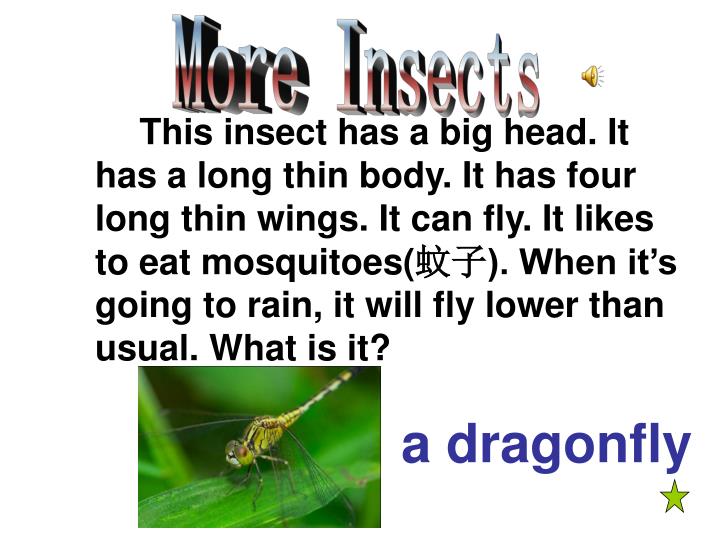At the top of the image, there's a heading in thick block letters with the top parts in light blue and the bottom parts in maroon, reading "More Insects." Below this, in smaller black text, it describes an insect with a big head, a long thin body, and four long thin wings. This insect can fly and likes to eat mosquitoes, with "wenzi" in Chinese characters in parentheses to clarify the term. The text also notes that when it’s going to rain, the insect will fly lower than usual. It ends with the question, "What is it?" To the right of this, in larger blue font, is the answer: "a dragonfly." Directly under the "y" in "dragonfly" is a small lime green star with five points. Below this text, there's an image of a lime green dragonfly resting on a bright green leaf. The image background is green and slightly blurry, emphasizing the dragonfly’s thin wings, distinct head, and pointed tail.